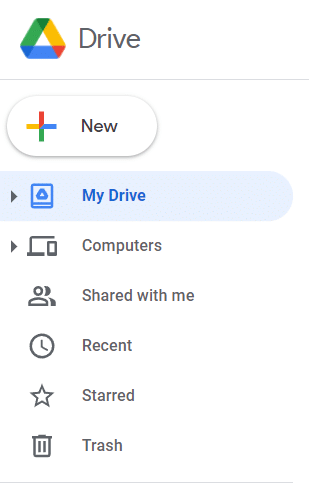In the image, we see a detailed screenshot of the top left-hand corner of the Google Drive platform interface. The prominent Google Drive logo, consisting of a triangular shape with segments colored blue, green, and yellow, is situated in the upper left-hand corner. Adjacent to the logo, the word “Drive” is displayed in clear, bold text.

Beneath the logo, there is a large button labeled "New," which users can click to create new files or folders. Directly below this button, a vertical list of six navigational options is visible. The first option, “My Drive,” is highlighted in blue, indicating it is currently selected. The subsequent five options, listed in descending order, include: “Computers,” “Shared with Me,” “Recent,” “Shared,” and “Trash.” These options provide users with various ways to access their files based on different criteria.

The entire interface is set against an all-white background, giving it a clean and minimalistic look. The screenshot effectively captures the essential navigation tools and layout of the Google Drive platform, emphasizing the organizational structure and user interface elements.